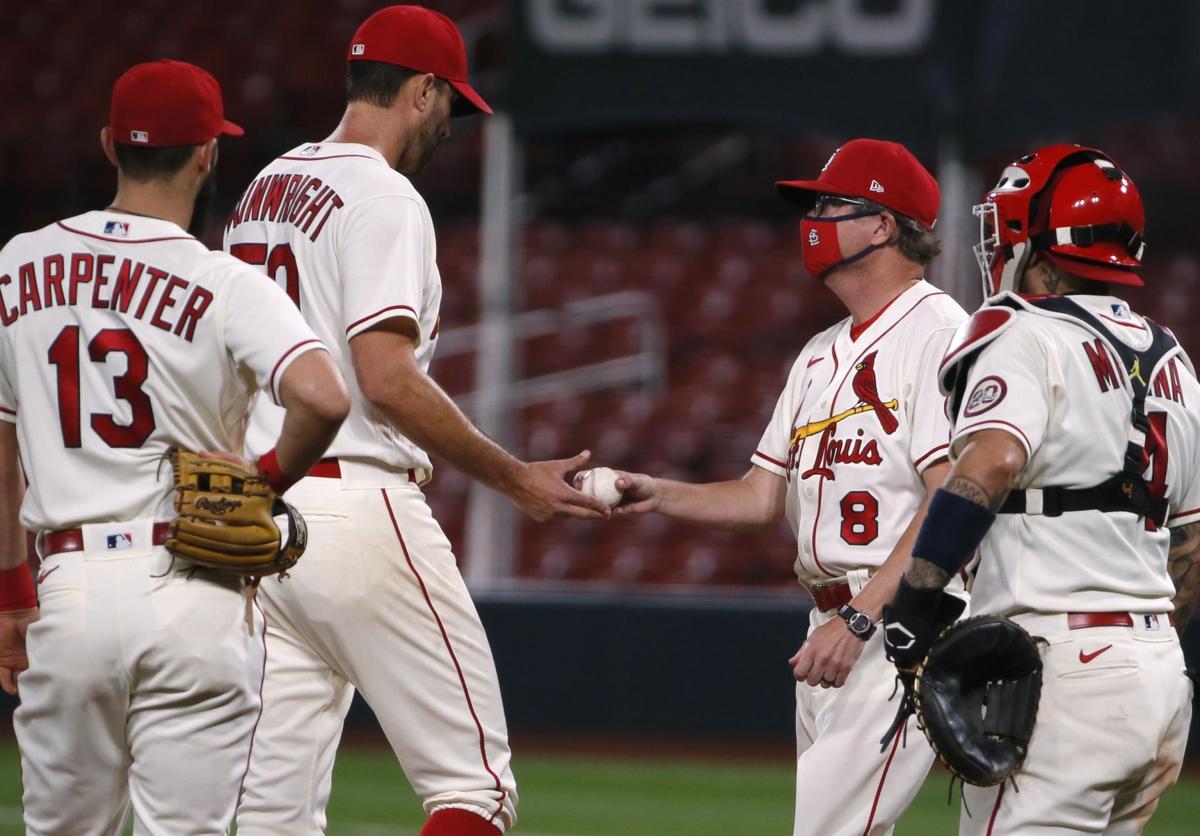In this vivid photograph taken on a brightly lit baseball field, four figures associated with the St. Louis Cardinals can be seen. Three of them are players and the other is an umpire, clad in distinctive red protective gear, a white outfit, and a black mitt. Positioned centrally, with his back turned, is Carpenter wearing the number 13 jersey. In an act that appears to symbolize a transition, Wainwright, the clearly visible pitcher, is handing a baseball to a tall Caucasian man wearing the number 8 on his jersey, who is likely the manager or coach. The scene captures a moment of interaction and focus, with another player standing nonchalantly with his hand on his hip. The background reveals the iconic red stadium seats of the Cardinals, somewhat blurred, suggesting an empty stadium. The colors in the image range vividly from white and red to green, yellow, dark blue, maroon, and black. This detailed, outdoor shot provides a clear and well-lit glimpse into a day on the field, emphasizing teamwork and the traditional elements of baseball.